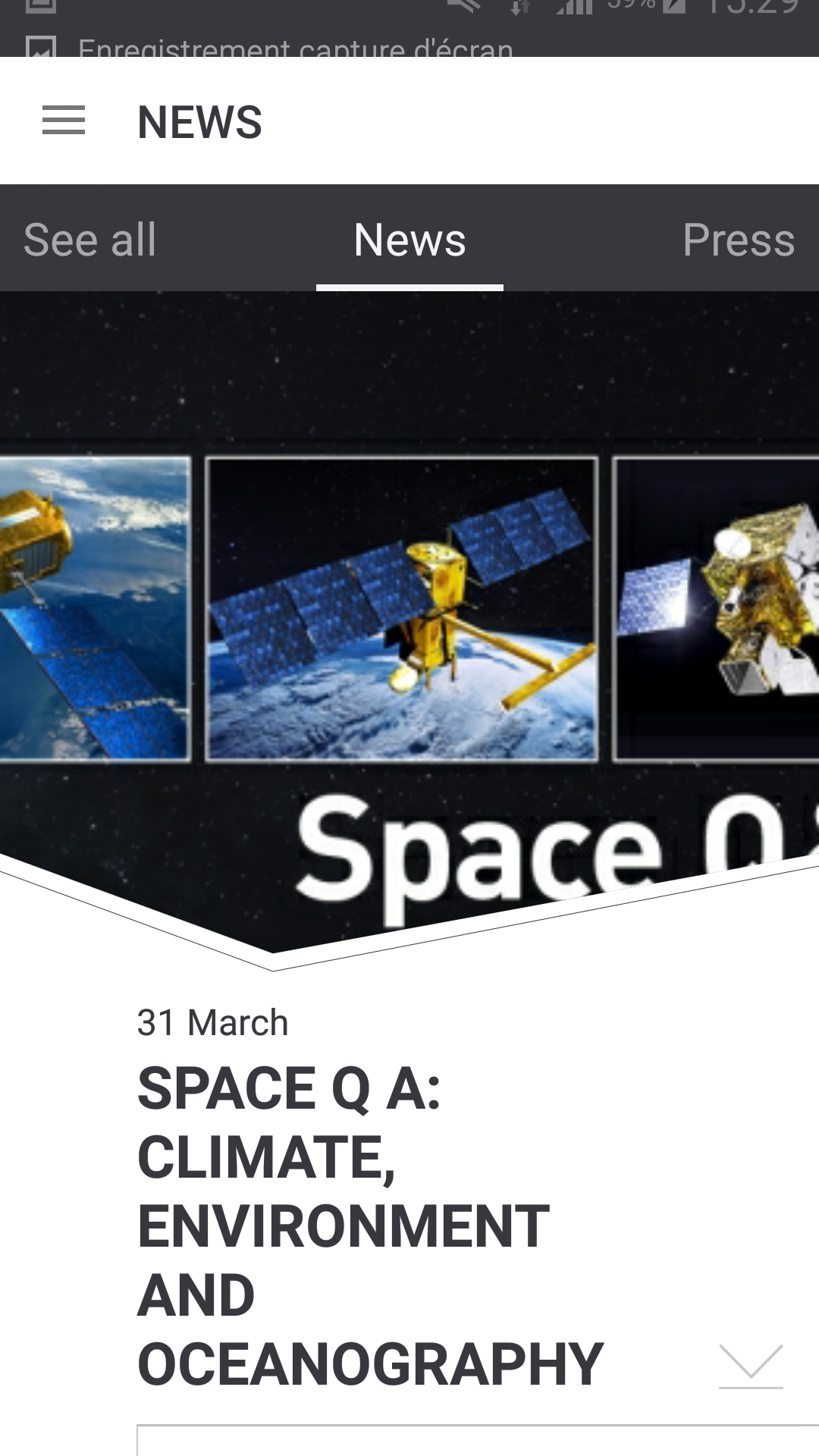An image captured from a cell phone shows an open news app, with the screen title in French reading "Enregistrement Capture de Crane." Below, there are three horizontal lines followed by the word "NEWS" in bold, capital letters. Under the header, there are options labeled "See All," "News," and "Press," with the "News" section selected. 

The main content appears to be related to space, possibly titled "Space Quest," though the full title is cut off. The screen displays multiple images in the news article, including a satellite orbiting above Earth and other objects in outer space. At the bottom of the screen, the date "31 March" is visible alongside an abbreviation "Space Q." This is followed by "Space A:" and topics related to "Climate, Environment, and Oceanography."